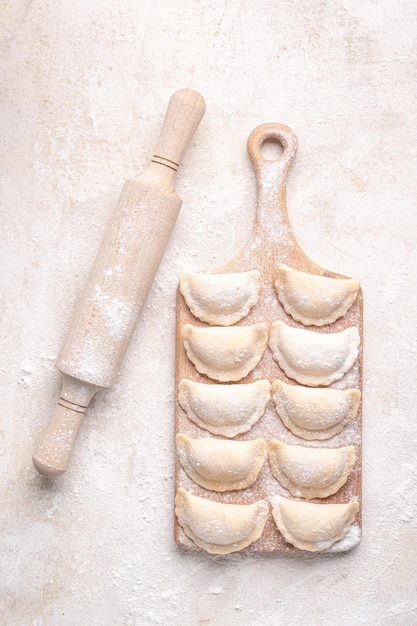In this overhead image, a baker's table is captured in a serene, flour-dusted scene. The pale beige, marbled countertop serves as the background, scattered with a light sprinkling of flour. To the left, a blonde wooden rolling pin, adorned with two gold stripes on each handle, lies at a slight 30-degree angle, covered in flour. Adjacent to it on the right, there is a blonde wooden cutting board featuring a top handle with a hole for easy gripping, also sprinkled with flour. 

Laid out neatly on the cutting board are ten crescent-shaped pastries, possibly dumplings, arranged in two vertical rows of five. These pastries are off-white with their edges crimped like pie crusts and appear partially baked, exhibiting slight browning on the edges. The delicate dusting of flour across the entire scene, from the countertop to the rolling pin and the pastries, adds a cohesive touch, highlighting a moment of preparation in a baker's craft.